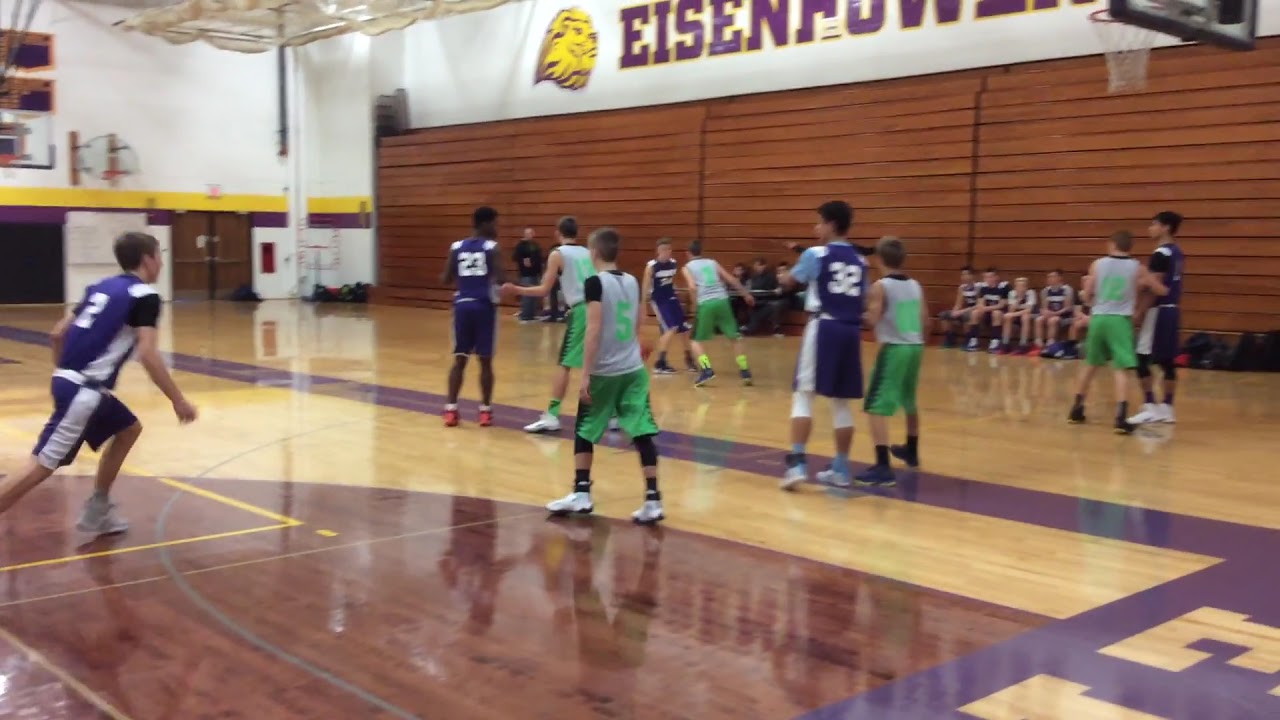This photograph captures an indoor high school gymnasium during a basketball game. The shiny hardwood floor, featuring alternating light and dark brown panels, and painted purple lines, reflects the vibrant activity on the court. Players are divided into two teams, with one team wearing blue and white uniforms and the other team in white shirts paired with green shorts. Centered on the court, the players are engaged in an intense game, while additional team members sit on the boundary benches. Above the closed wooden bleachers, the white walls display a banner adorned with a red, gold-outlined logo of a lion's head and part of the name "Eisenhower" in bold red text. This setting, likely a high school gymnasium, showcases not only the competitive spirit of the game but also the meticulous indoor environment with its distinctive color palette and well-maintained features, including visible basketball hoops at both ends of the court.